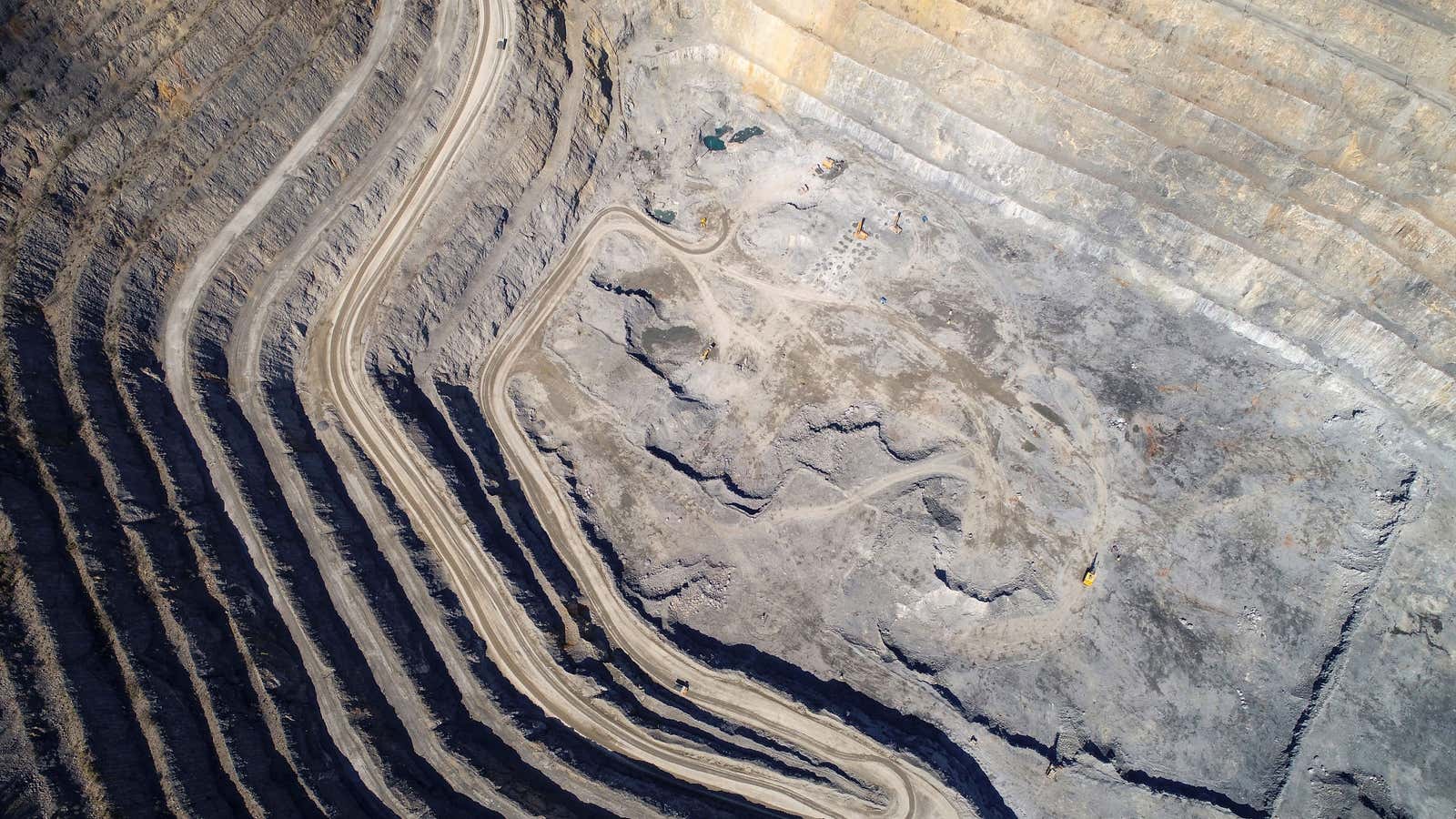This top-down image showcases a vast, terraced surface mine, often referred to as a strip mine. The horizontal, rectangular photograph reveals a complex network of ridges resembling shelves of rock, which have been meticulously carved out to allow trucks to descend to deeper levels of the mine. The terrain is predominantly gray, interspersed with darker patches, indicating the possible presence of some type of ore being extracted. The terraced layout is especially prominent towards the left and bottom with shadows creating a gradient effect, making the deeper parts appear almost black. Conversely, the upper right section, bathed in sunlight, reveals the stratified layers more distinctly. The landscape is entirely barren, devoid of any vegetation, enhancing the stark, industrial nature of the scene. Although the mine appears deserted at the moment, there may be tiny vehicles or carts scattered within, so small they are barely discernible.